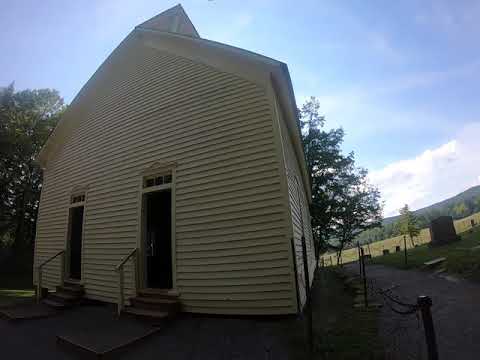The image depicts an older, white clapboard building with two parallel entrances, each featuring three steps and handrails. The fisheye lens captures mainly one side of this two-story structure, highlighting its plain, unmarked exterior which could suggest it's a side entrance. The building evokes the architecture of a church or a schoolhouse and is set in a rural location adorned with trees and a few scattered clouds in a blue sky. In the background, an open field contains gravestones, hinting that the field might be a churchyard. A small gravel path runs alongside the building, bordered by posts with chains likely used to guide or restrict visitors. The understated design, devoid of any signage or religious symbols, adds an element of mystery to its exact purpose, be it for tours or a functional space within a community.